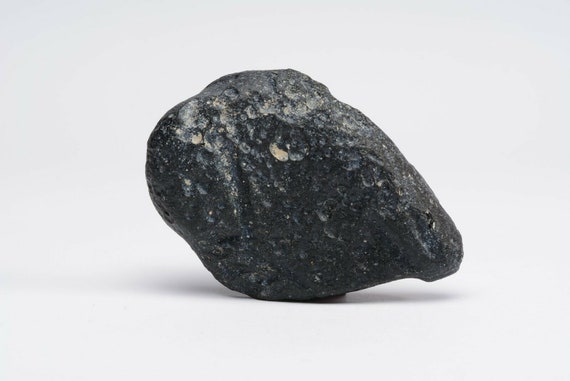This image features a black rock positioned centrally against a stark white background. The rock, which appears somewhat oval but thins on the right side, has a striking resemblance to a lamb's or sheep's head due to a distinctive white mark resembling an eye on its upper right side. The surface of the rock is mostly smooth with a few indentations, some revealing a subtle yellowish hue. A small shadow beneath it spans from gray to black, emphasizing its three-dimensional presence. The rock's detailed texture includes tiny craters and a chipped section on one side.